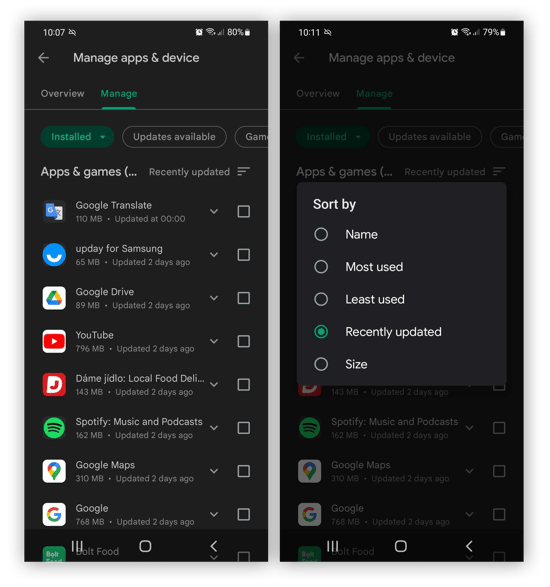The image comprises two side-by-side screenshots of an Android smartphone, captured at 10:07 AM. The device is connected to a Wi-Fi network and shows two bars of cellular service with an 80% battery life.

The left screenshot displays the "Manage Apps and Devices" menu with the "Manage" tab selected and filtered for "Installed" applications. Below the headings "Apps and Games," the apps are sorted by "Recently Updated," and the following applications are listed:

1. **Google Translate**: 110 MB, updated today.
2. **UDPay for Samsung**: 65 MB, updated 2 days ago.
3. **Google Drive**: 89 MB, updated 2 days ago.
4. **YouTube**: 796 MB, updated 2 days ago.
5. **Dame Judeo, Local Food Delivery**: 143 MB, updated 2 days ago.
6. **Spotify Musics and Podcasts**: 162 MB, updated 2 days ago.
7. **Google Maps**: 310 MB, updated 2 days ago.
8. **Google**: 768 MB, updated 2 days ago.

Each app is displayed with the standard Android application thumbnail, and none are currently selected.

The right screenshot shows the same "Manage Apps and Devices" page. This time, the "Sort by" dropdown menu is open, obscuring most of the page. The menu offers the following sorting options: 

- Name
- Most Used
- Least Used
- Recently Updated
- Size

The option "Recently Updated" is selected, indicated by a green bubble next to its entry. The other options also have bubbles next to them, though they remain unfilled, unlike the green-filled bubble next to "Recently Updated."